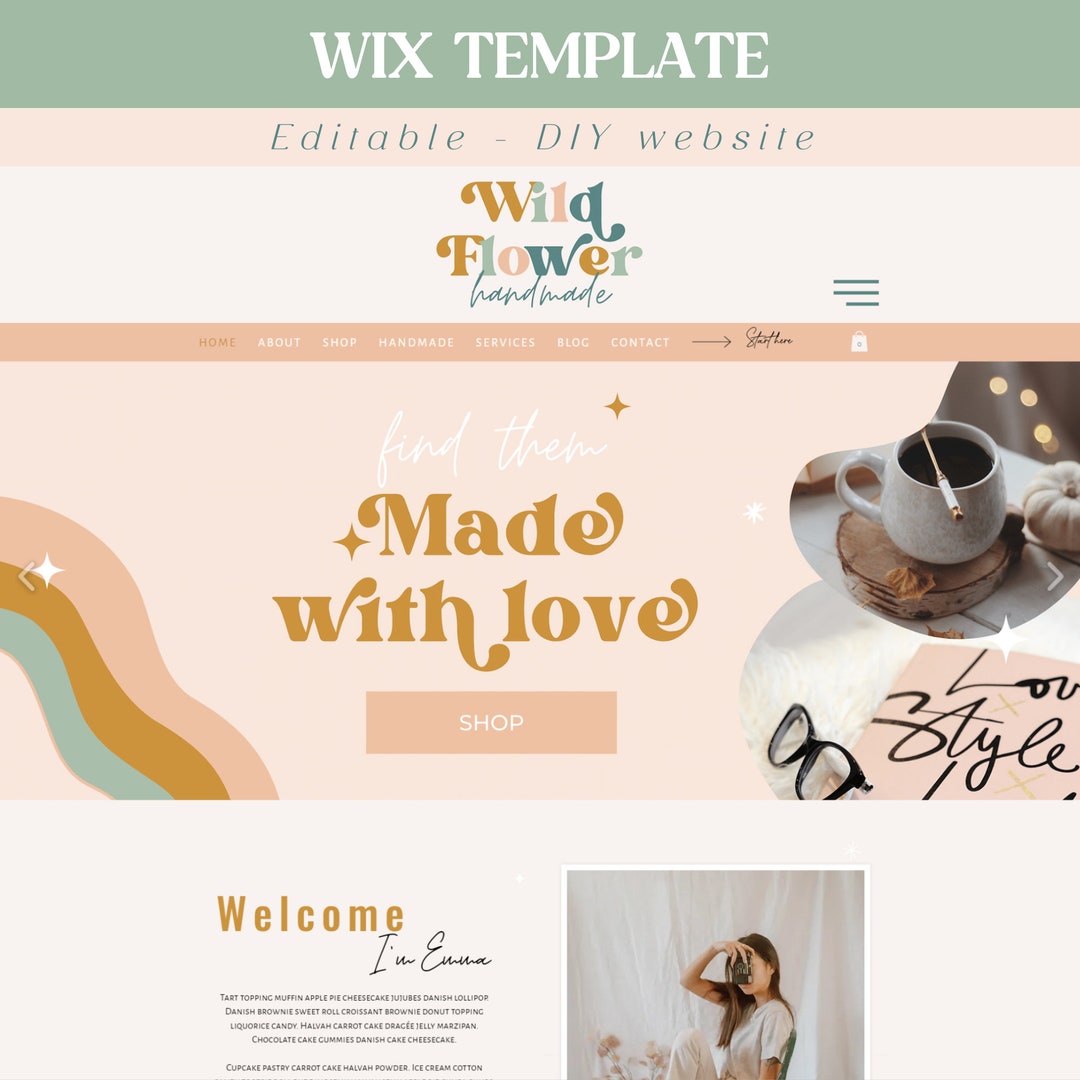This is a detailed marketing flyer for a DIY website template from Wix, featuring the "Wildflower Handmade" design. The header prominently displays "Wix Template" in white font against a green background. Below it, "Editable DIY Website" is highlighted in a smaller, artsy font on an off-white band. The title "Wildflower" stands out in a multicolored, ornate font using shades like brown, light blue, pink, and dark blue, complemented with cursive text reading "handmade." The flyer has a chic, pink-themed background, adding a soft aesthetic touch.

The central part of the flyer includes actionable text: "Find These Made With Love," accompanied by a clickable "shop" button. To the right, there's a cozy setup with a coffee cup on a coaster, a honey dipper resting across it, and a pair of reading glasses, suggesting a blend of comfort and creativity. In one corner, a portrait of a woman identified as Emma holds a camera, appearing to take a photo of the viewer, adding a personal touch. Below this image, "Welcome, I’m Emma" introduces her, likely followed by a small bio in fine print that emphasizes her role and story behind the brand.

Navigation links labeled "home, about, shop, handmade, services, blog, contact" are situated below the primary header, aligning with website features. The blended details point towards this being a promotional snapshot emphasizing ease of use and customization for small business owners or creatives looking to design their websites with Wix.